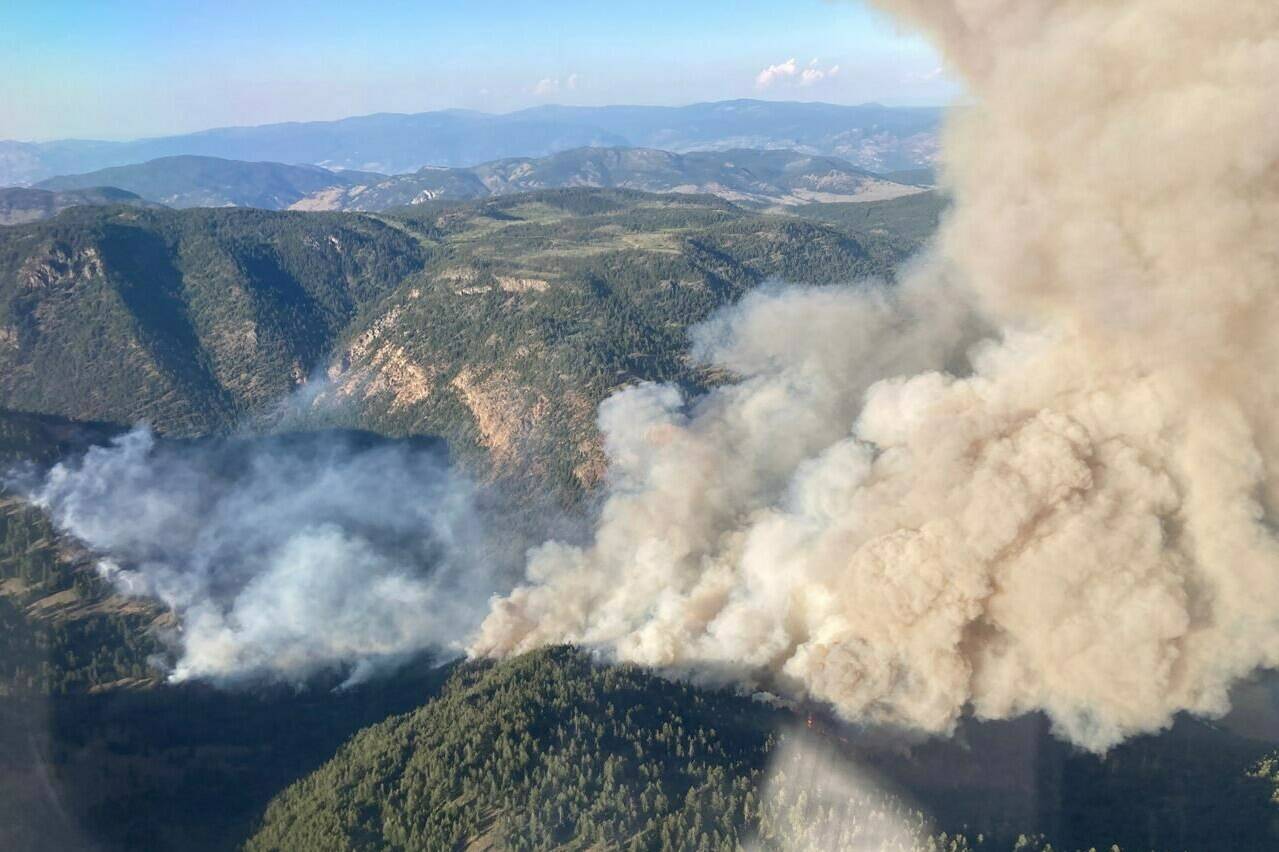The image is an aerial photograph capturing an expansive view of a mountainous region covered in a dense forest. The forest is engulfed in a wildfire, evident from the plume of black to grayish-brown smoke billowing upward. The smoke widens toward the bottom, emanating from the forested valleys directly below, and gets more dirty and brownish as it rises. There are noticeable patches of green trees blanketing the rolling hills and mountains, which appear to maintain a consistent height without becoming extremely tall. A small, orange flame is visible at the base of the smoke, accentuating the severity of the fire. The photograph seems to be taken from an aircraft, as evidenced by the reflection of possibly a plane or helicopter window. The far background reveals a contrast of serene blue sky and white clouds, juxtaposed with the worrisome haze caused by the fire. The scene captures the dramatic impact of the wildfire amidst the lush green landscape, with the presence of shadows adding depth and definition to the terrain. It appears to be summer, and the location might be somewhere in the western United States, characterized by what looks like pine or evergreen trees.